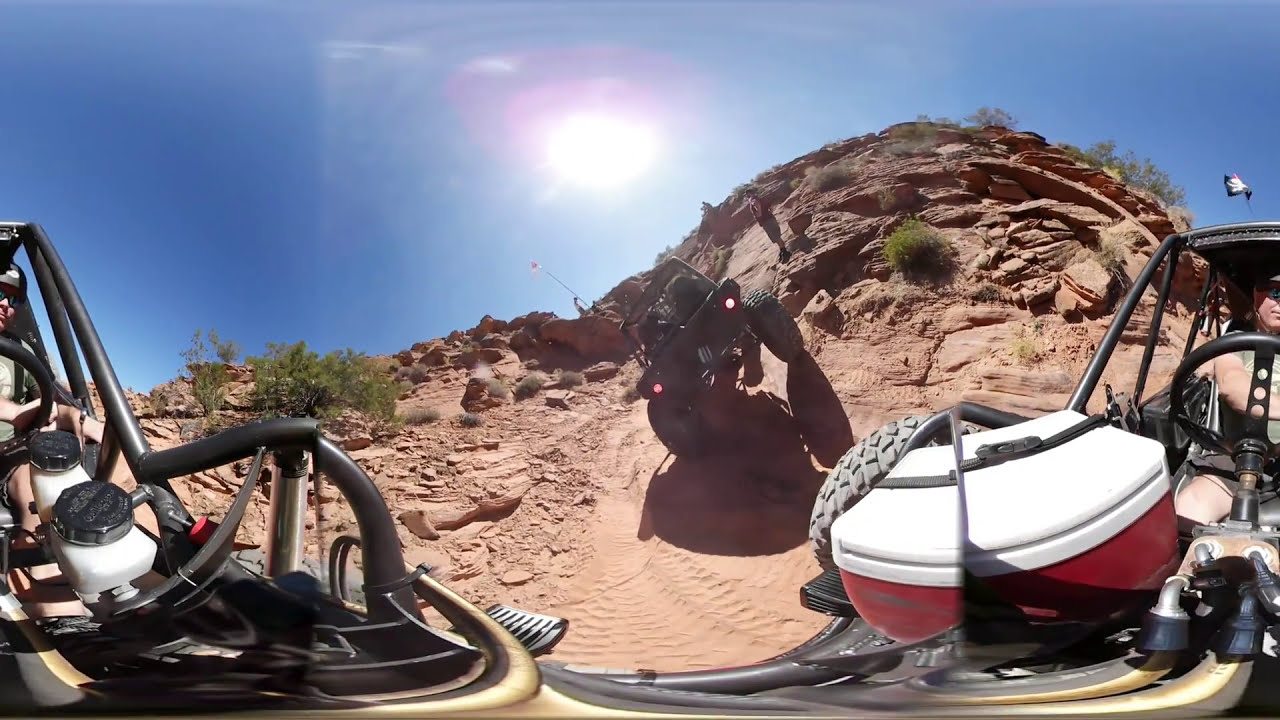In this image, three off-road ATVs traverse a rugged, rocky desert terrain on a bright and sunny day. The clear blue sky forms a striking backdrop. One vehicle, driven by a man, is positioned to the right, moving forward, while another dark vehicle is centered, driving away from the viewer. A third ATV is tilted on its side, highlighting the challenging and uneven landscape. The terrain is dotted with rocks, gravel, and sparse bushes, adding to the arid, rugged ambiance. A notable feature is a red cooler with a white lid in one of the vehicles. Additionally, a person clad in a red shirt, knee-length shorts, and black tennis shoes is seen standing on a rock cliff, overlooking the scene. The bright sun casts sharp shadows, emphasizing the hilly and desolate environment.